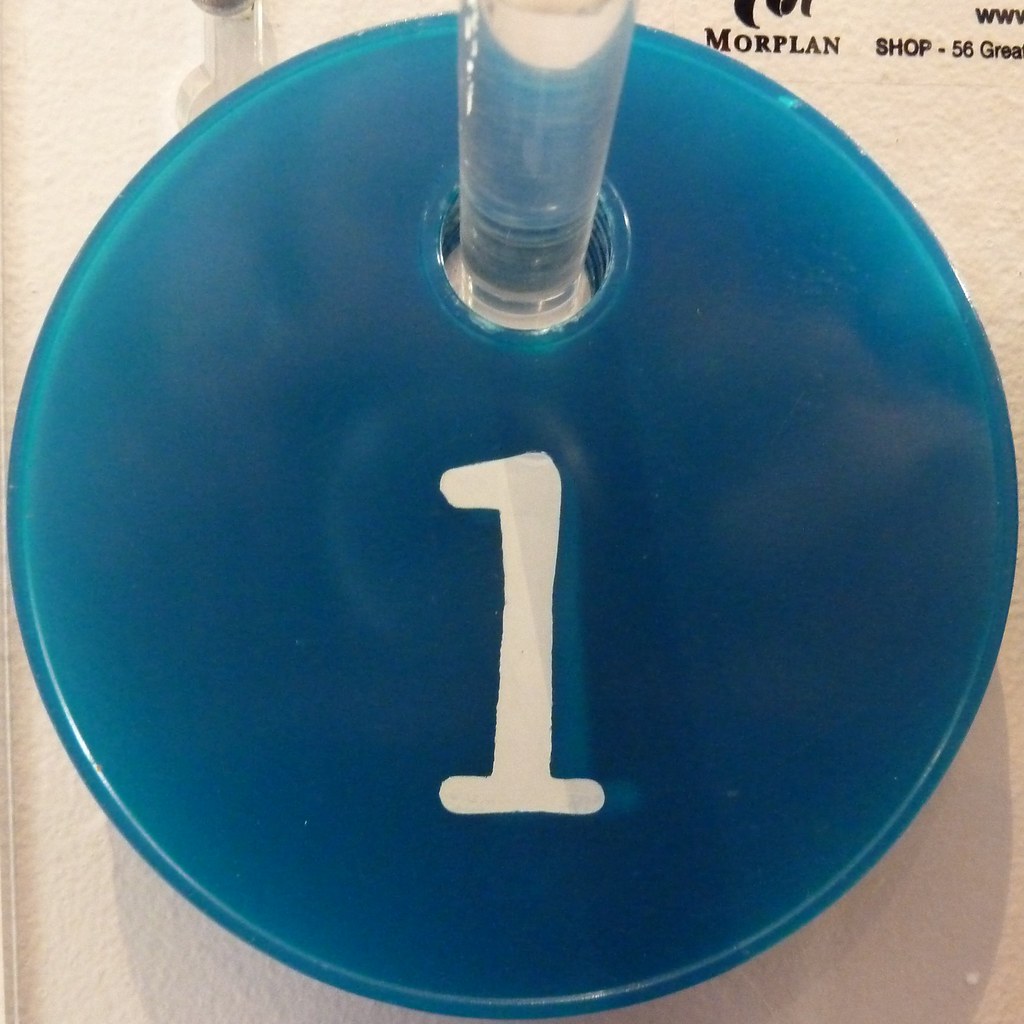The image is a photograph showcasing large, semi-transparent blue discs made of acrylic plastic, each having a distinct white number painted on them—the prominent disc in the front displays a '1', while the one behind it features a '9'. The discs, which have holes in their centers, are stacked on a clear acrylic peg that is mounted on a white-textured wall. In the top right corner, black text in all caps reads "MORPLAN SHOP-56GT WW." The discs appear to rest on a light tan or beige surface. The main colors in the image are dark brown for the text, light tan, blue, and white.